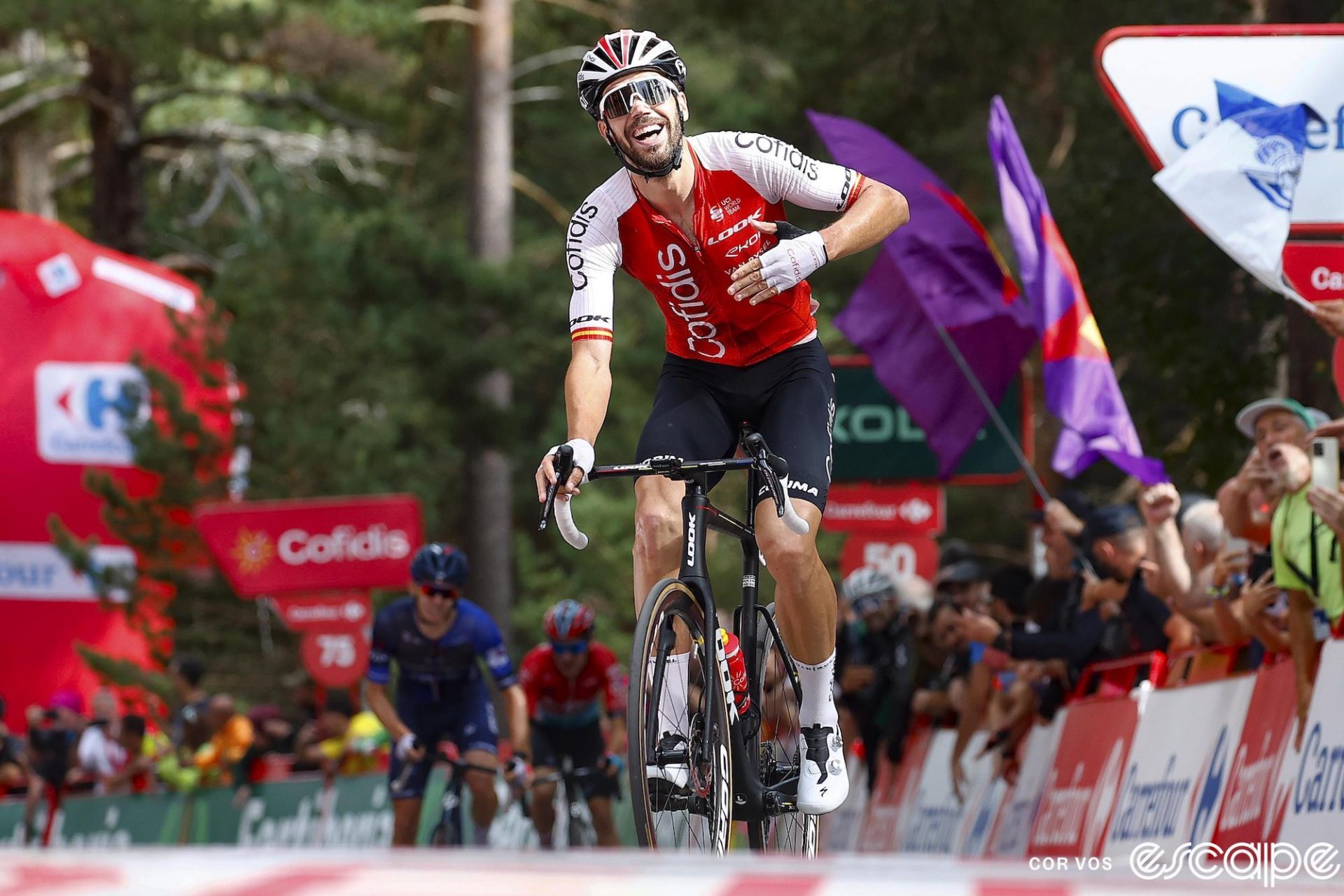The photograph captures the exhilarating moment at what appears to be the finish line of a bicycle race, with numerous signs and billboards indicating a competitive event. The central figure, a seemingly victorious and jubilant cyclist, is adorned in a distinctive red and white jersey with "Cofidis" emblazoned on it. His outfit is complemented by black bike shorts, white biking shoes, white crew socks reaching his calves, and a white and red helmet with a ridged design typical for cycling gear. The cyclist also sports black sunglasses with white frames and fingerless gloves. His right hand grips the handlebars of his black road bike, while his left arm is raised in a celebratory gesture.

Lush green trees with prominent brown branches form a picturesque backdrop, suggesting a summer or late spring setting. Around the cyclist, an enthusiastic crowd behind red and white barricades waves various flags, including some purple ones with red, yellow, and white, and another blue and white flag with an indistinct emblem. Surrounding the scene are numerous billboards with the “Cofidis” brand and other advertisements, partially obscured by the motion of the crowd's flags. In the distance, there is a large red inflatable structure adorned with more ads.

Flanking the main cyclist are two other riders donning blue and red uniforms, each with blue helmets, and devoid of the exuberance on the face of the lead cyclist, implying they have not won. The entire scene is imbued with the energy and excitement of the race's conclusion, accentuated by a red and white striped finish line towards the bottom of the image, hinting at the dramatic culmination of the competition.